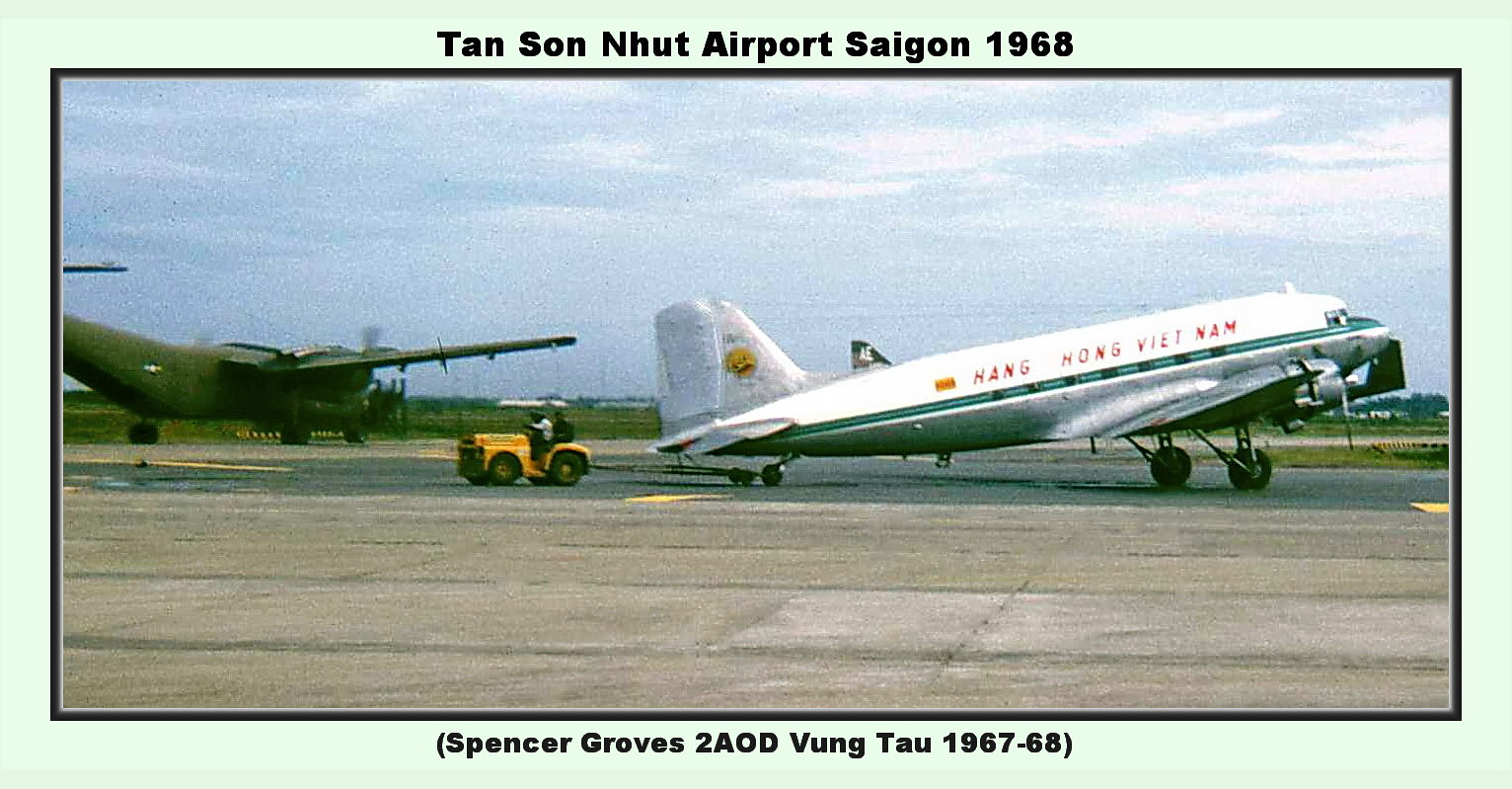The image depicts a photograph bordered by a green outline, with a darker green thin line running inside the border. At the top, bold text reads "Tan Son Nhat Airport, Saigon, 1968," and at the bottom, in parentheses, it says "Spencer Groves II AOD, Vung Tau, 1967-68." The scene captures an airport runway where two large airplanes are parked on a cement area. The airplane on the right side, viewed from the side, is predominantly white with a green stripe running the length of its body, and carries red lettering saying "Hang Hong Vietnam" above a blue stripe. This white aircraft is connected to a yellow tractor, which appears to be towing it, and two people are visible inside the tractor. The airplane on the left is facing away from the camera, showcasing its army green color and propellers that seem to be in motion. The sky in the background is clear blue with a few white clouds, completing the detailed vintage airport scene from 1968.